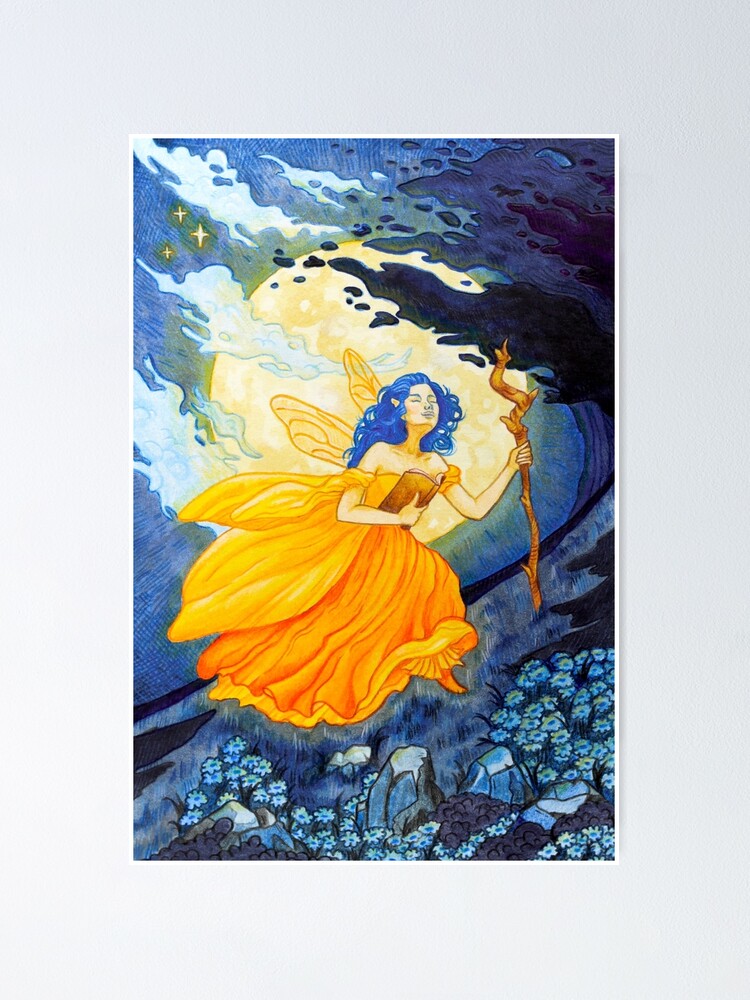The detailed image displays a fantasy scene of a female fairy with long, bright blue hair flying across a flower bed of blue flowers. She wears a flowing yellow-orange dress and has slightly translucent yellow wings. In one hand, she holds a spiny wooden staff, and in the other, she cradles a book against her chest. The scene is illuminated by a massive full moon, partially covered by both white and dark clouds, making the night sky magical and surreal. She floats gracefully in front of the moon, casting a serene and enchanting aura over the dreamlike landscape, which includes a hillside dotted with blue daisy-like flowers and a couple of rocks, hinting at a fantastical world below her. The background, though white, complements the ethereal essence of the artwork, seamlessly blending elements that could be depicted underwater or on land. The fairy's eyes are closed, enhancing the mystical tranquility of the scene.